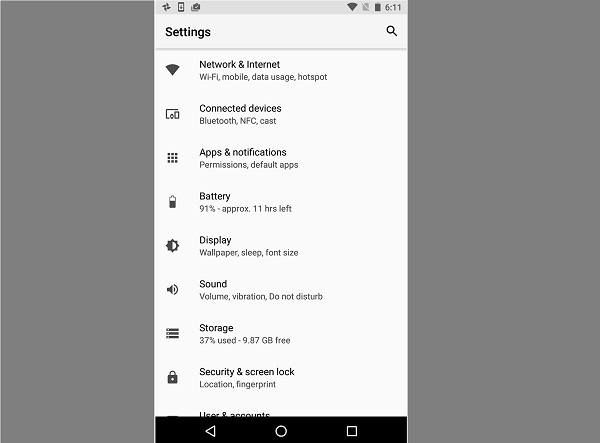The image displays a mobile phone screen currently in the settings menu. The visible sections include:

1. **Network & Internet**: For managing Wi-Fi, mobile data usage, and hotspot settings.
2. **Connected Devices**: Options for Bluetooth, NFC, and casting (screen mirroring).
3. **Apps & Notifications**: Where you can manage app permissions, default apps, and notifications settings.
4. **Battery**: Indicating approximately 11 hours of battery life remaining.
5. **Display**: Configurable options such as wallpaper, sleep timer, and font size.
6. **Sound**: Settings for volume, vibration, and Do Not Disturb mode.
7. **Storage**: Showing that 37% is used, with 9.87 GB free.
8. **Security & Screen Lock**: Indicated by a padlock icon, with options for location and fingerprint security.

All settings appear closed, organized by section to allow the user to customize various aspects of their device.